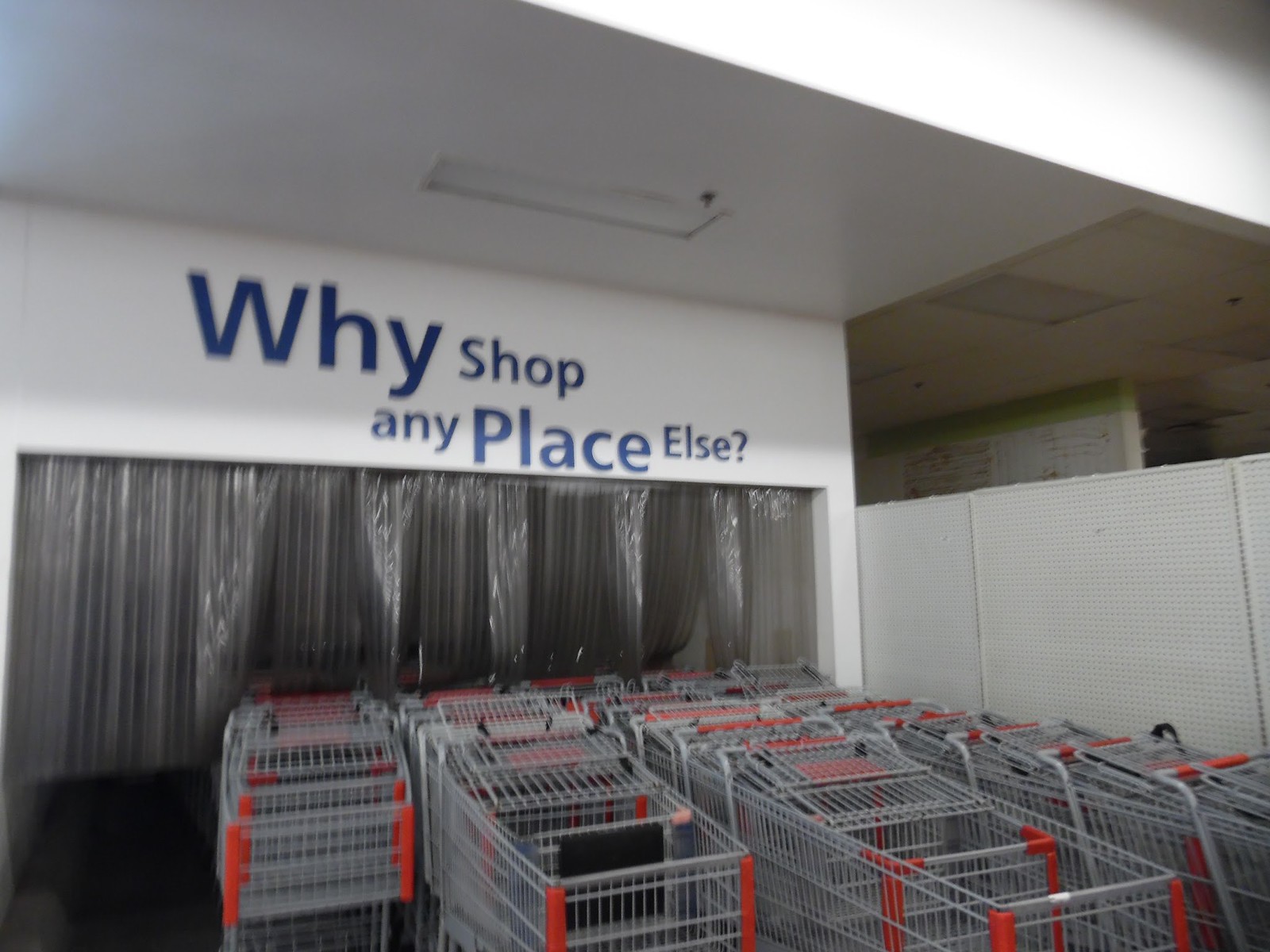The image depicts the interior section of a typical supermarket entrance area designated for storing shopping carts. This specific area features a white ceiling and white walls. A noticeable feature is the cutout section of the wall, filled with somewhat transparent plastic flaps, allowing shopping carts to be pushed through from the outside of the building. The shopping carts are uniformly gray with red handles and red edging.

On the wall above the cart station, there is a prominent blue text reading, "Why shop any place else?" followed by a question mark. Above this, the white ceiling has a cutout, potentially accommodating a vent or fan, contributing to the airflow in the space. In the upper right corner, another cutout opening is visible on the wall, revealing additional walls behind it and what seems to be another vent in the ceiling area.

The overall quality of the image is shadowy and of low resolution, making finer details hard to discern, but the layout and key features are still identifiable.